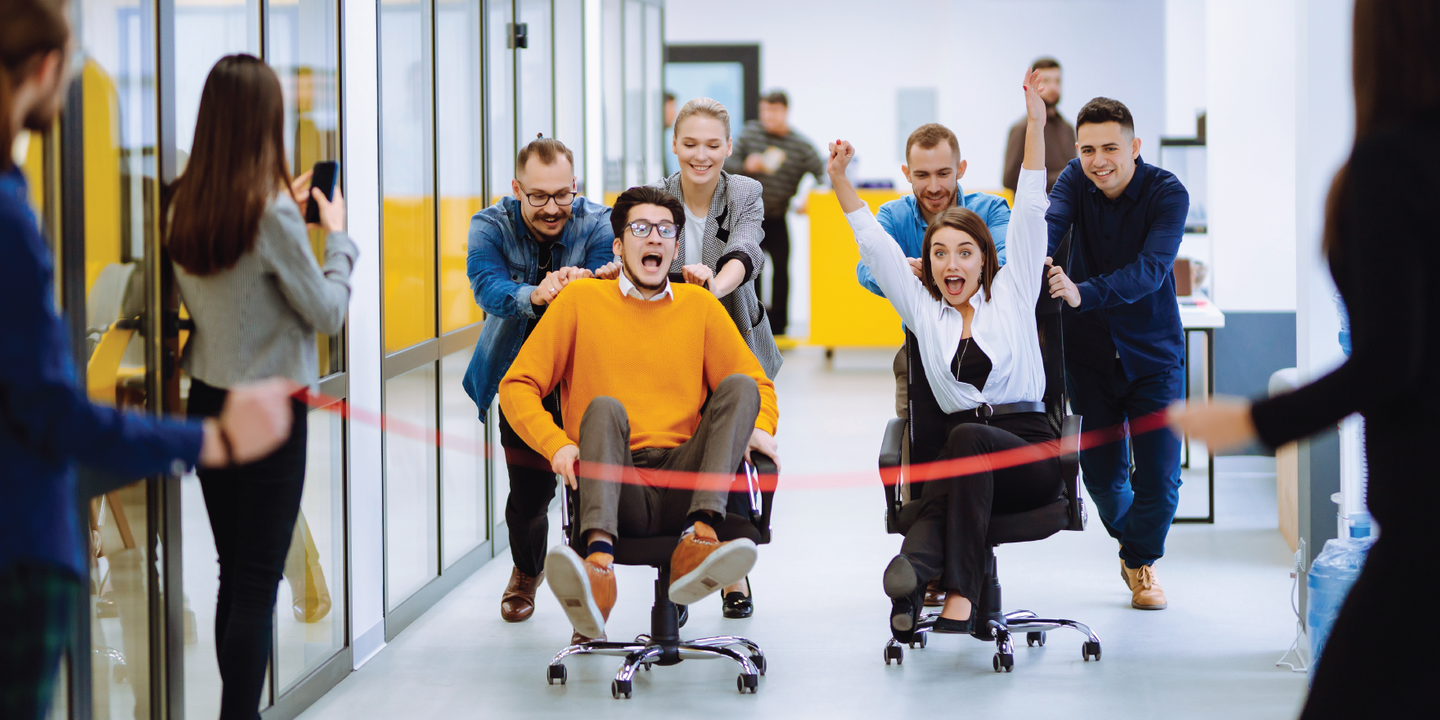In this vibrant and lively office scene, a chair race takes center stage in a predominantly white modern workspace characterized by white floors, walls, and glass-panelled corridors. In the foreground, two competitors— a man in a yellow sweatshirt and light brown pants, and a woman wearing a white blouse with a black under blouse and dark brown pants— are seated on rolling office chairs, clearly reveling in the excitement. The man's feet are lifted off the ground in exhilaration, while the woman's arms are jubilantly raised as if in anticipation of a victory. 

Each racer is being enthusiastically pushed by two colleagues towards a finish line marked by a red ribbon. This ribbon is held by a man in a blue jacket to the right and is slightly out of focus as it extends to another person on the left. Surrounding them, an energized crowd of about ten people, some of whom are blurred and standing against the far wall, cheer and capture the moment with their phones. One particularly engaged onlooker actively films the race from the left side of the corridor. This joyful event seems to be an office-sanctioned celebration or party, as everybody is visibly happy and participating in the fun.